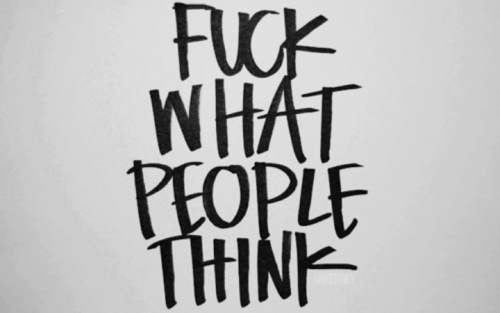The image displays a simple, attention-grabbing sign that one might post on social media platforms like Instagram or Facebook. It features a blank white background with four lines of black text, each line containing one word in all capital letters: "FUCK" on the top line, "WHAT" underneath, followed by "PEOPLE," and "THINK" at the bottom. The letters appear to be handwritten with a marker, giving them an imperfect and human touch. The text as a whole is bold and sharp, though not precisely aligned. The U in "FUCK" lacks the right vertical line, resembling more of an unfinished curve. The K in the same word has an unusually elevated right leg, almost horizontal. Additionally, the final E in "PEOPLE" has a bottom leg that curves upward at a 45-degree angle, deviating from the usual straight line. Overall, the sign’s message is direct and unfiltered, emphasizing a carefree attitude toward others' opinions.